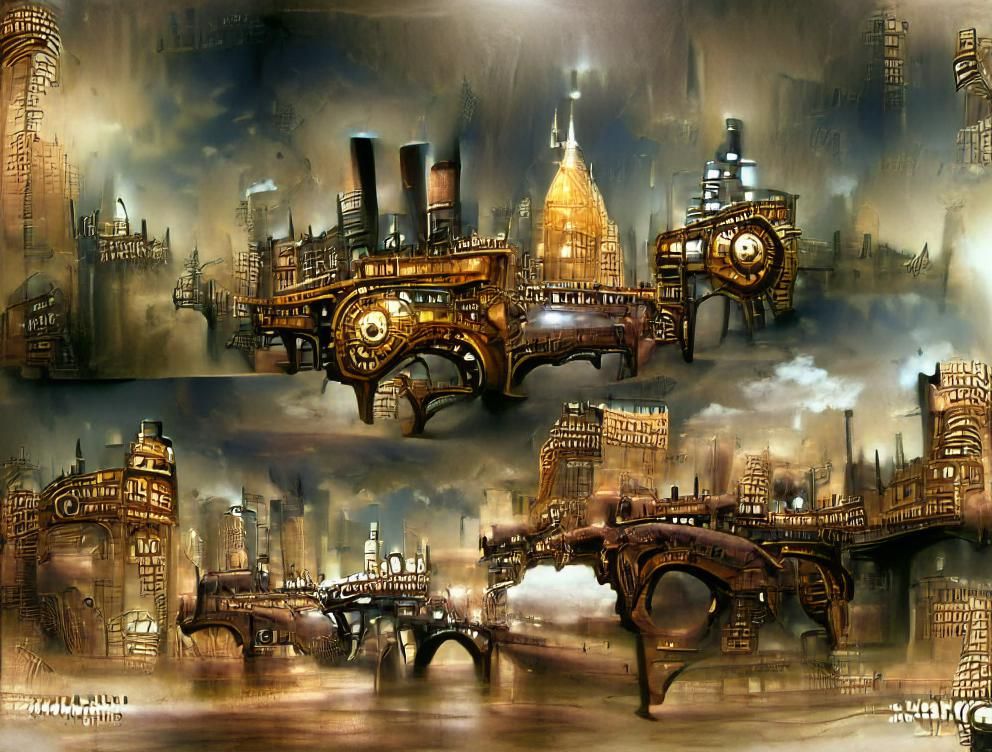In this up-close, abstract image, a fantastical steampunk cityscape unfolds before the viewer. Inspired by the architectural essence of London, the city is depicted with elongated, distorted skyscrapers and broken bridges that stretch in various directions, creating an eerie sense of surrealism. The foreground reveals what could either be slick roads or water, with reflections adding to the ethereal quality of the scene. The absence of humans contrasts with the abundant lights glowing from within and around the structures, casting a golden hue amidst the predominantly brown and dreary palette. Indescribable shapes abound, with notable features including a well-lit building with a steeple in the center, and a trio of smokestacks piercing the sky which is dense with fog and clouds. The overall atmosphere exudes a sense of pollution and melancholy, heightening the intricate beauty of this fantastical cityscape.